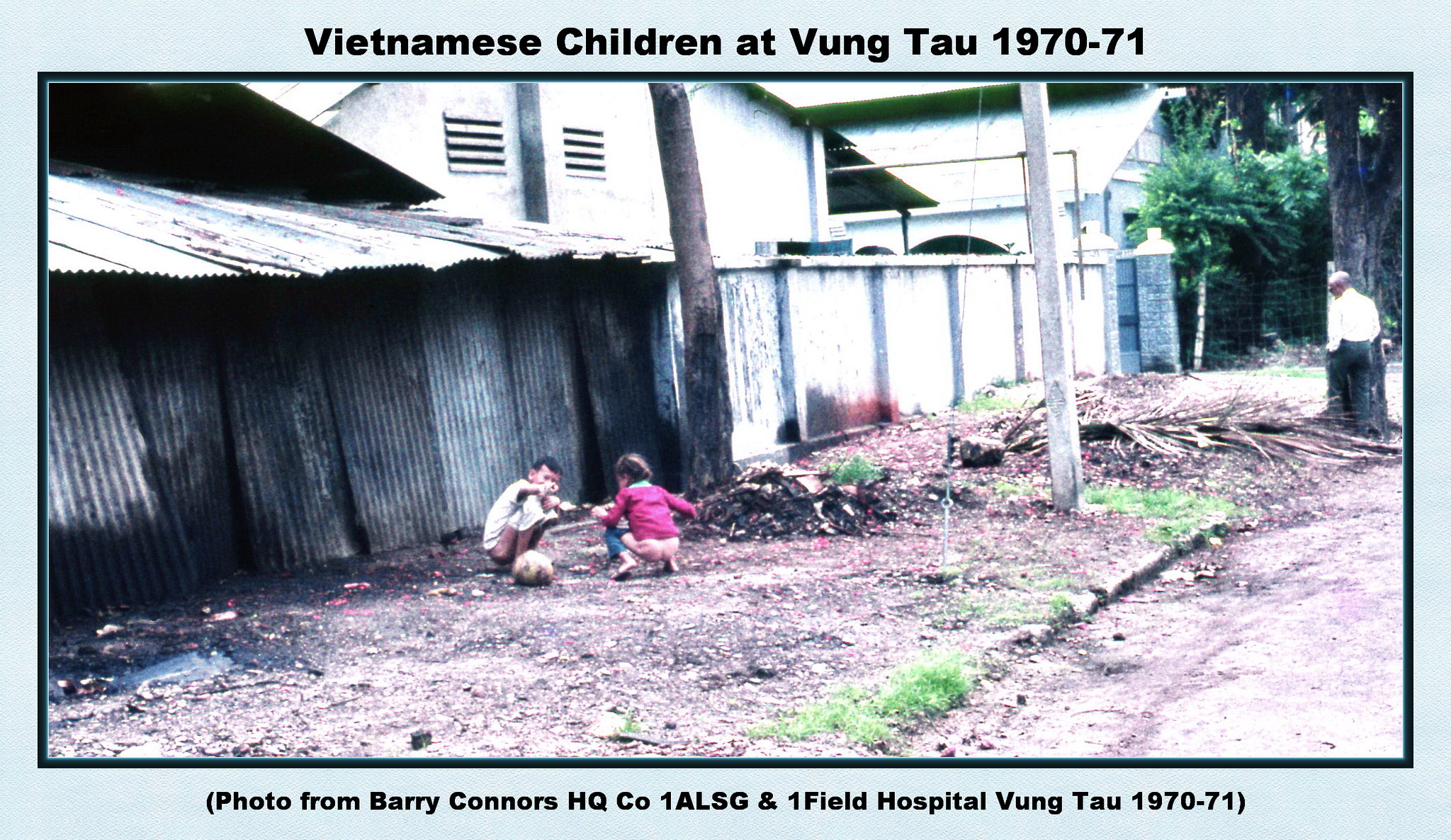A historical photograph taken by Barry Connors during 1970-71 in Vung Tau, Vietnam, featuring two young Vietnamese children, possibly siblings, approximately under eight years old, playing in an open field. The girl, dressed in a vibrant hot pink or magenta jacket, and the boy are both kneeling beside a ball, appearing engrossed in a game amidst rudimentary, tin-roofed shanties with visible burn marks. An elderly man, clad in a white button-down shirt and black slacks, stands in the background near a tree, observing the children, possibly their guardian. This image is marked with the text "Photo from Barry Connors, HQ CO 1 ALSG and 1 Field Hospital Vung Tau, 1970-71."